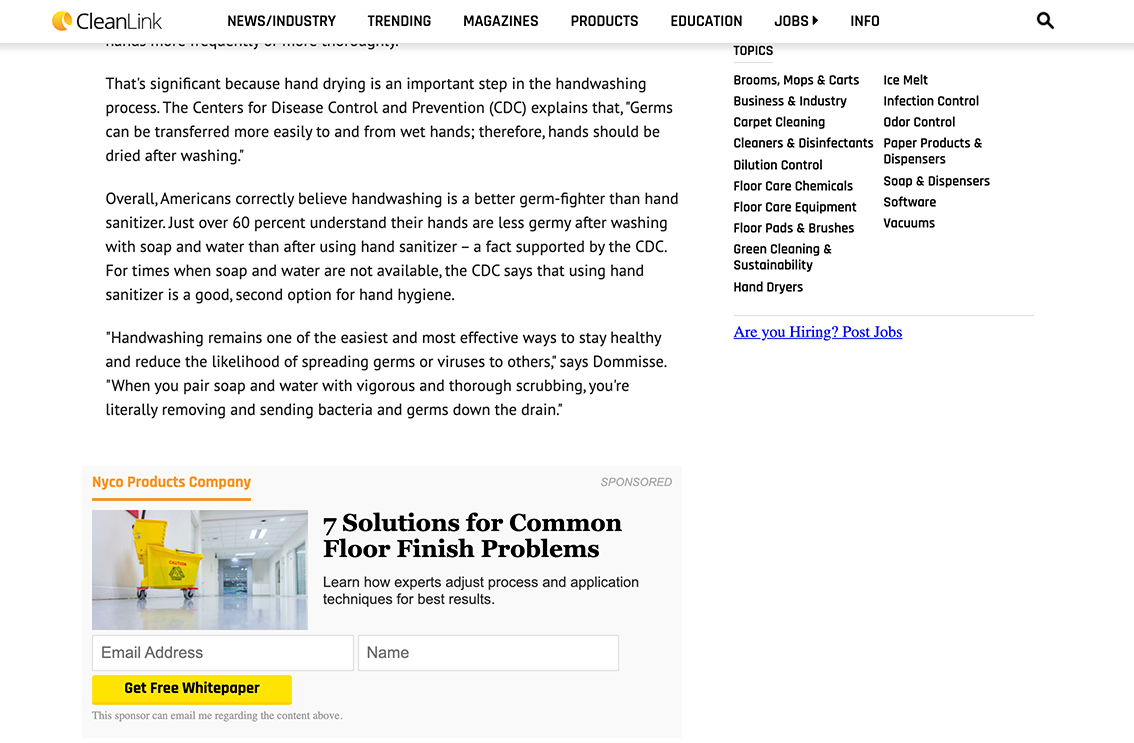The webpage showcases Clean Link, identifiable by its distinctive logo on the top left—a dynamic orange swoosh that transitions from narrow to thick and changes in shade before narrowing again. Next to the logo, the site title "Clean Link" is displayed with "clean" in bold black text and "link" in regular black text. Further along the header is a menu bar with several options displayed in small, bold, capitalized black text: "NEWS / INDUSTRY," "TRENDING," "MAGAZINE," "PRODUCTS," "EDUCATION," "JOBS," with an adjacent right-pointing arrow for the jobs section, and finally, "INFO." A magnifying glass icon, angled to the left, indicates the search functionality near the end of the menu.

Below the header, an article begins, emphasizing the importance of hand drying as part of the hand washing process. The first paragraph highlights the significance, citing the Centers for Disease Control and Prevention (CDC): "Germs can be transferred more easily to and from wet hands. Therefore, hands should be dried after washing."

To the right of the article, a list of topics is presented in black text, covering categories such as "Brooms, Mops, and Carts," "Business and Industry," "Carpet Cleaning," "Cleaners and Disinfectants," "Dilution Control," "Floor Care Chemicals," "Floor Care Equipment," "Floor Pads and Brushes," "Green Cleaning and Sustainability," "Hand Dryers," "Ice Melt," "Infection Control," "Odor Control," "Paper Products and Dispensers," "Soap and Dispensers," "Software," and "Vacuums."